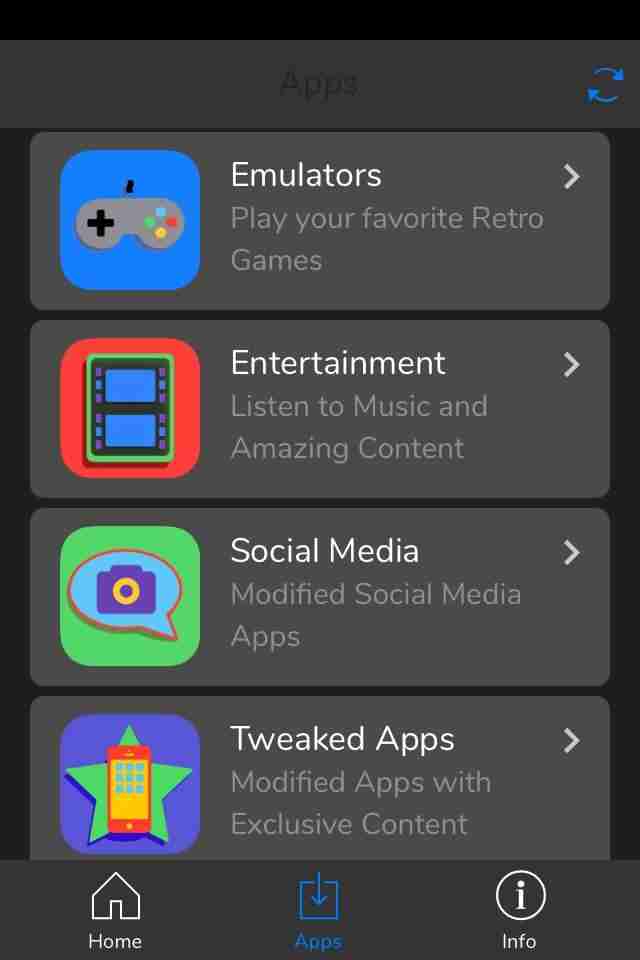**Detailed Caption:**

The image is a screenshot of a mobile application interface featuring a sleek, dark-themed design. The main background is black. 

At the top of the screen, there's a thin, black stripe followed by a medium gray or dark gray header. Within this header, slightly blurry and very dark gray text reads "Apps". Positioned at the far right of the header is a blue refresh icon consisting of two arrows: one pointing down and to the right, and the other pointing up and to the left.

Below the header, against the black background, there is a list of options presented in rectangles with dark gray backgrounds and rounded corners. Each option includes an icon on the left side with a colored background and a corresponding icon in the center. Next to each icon are a white title and a medium gray description.

1. The first option has a blue background with a gray game controller icon. The title "Play your favorite retro games" is displayed in white.
2. The second option features a red background with a filmstrip icon. Its title reads "Entertainment", and the description states "Listen to music and amazing content".
3. The third option has a green background with a blue speech bubble icon containing a purple camera. The title is "Social Media" with the description "Modified social media apps".
4. The fourth option boasts a purple background with a green star, and within the star is a red cell phone with a yellow screen. It is titled "Tweaked Apps" and described as "Modified apps with exclusive content".

Each of these dark gray rectangles has a white arrow pointing to the right in the top right corner, indicating the ability to navigate further into each option.

At the bottom of the screen, there is a dark gray footer featuring three icons labeled as follows:
- The first icon is a house, labeled "Home".
- The second icon, highlighted in blue, is a square with an arrow, labeled "Apps".
- The third icon is a circle containing an eye, labeled "Info".

This clear and detailed interface design ensures the user can easily navigate and understand the purpose of each section.